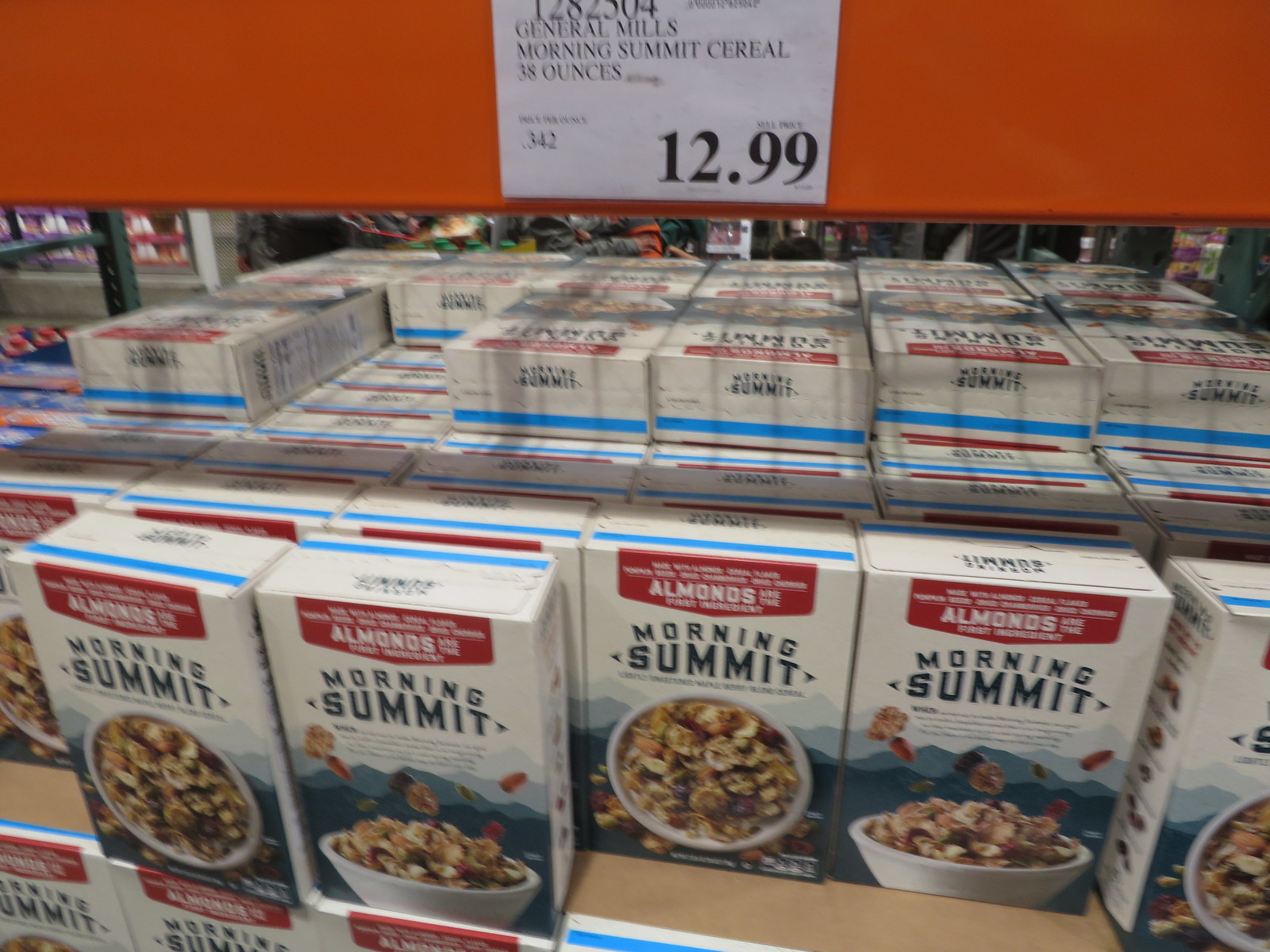This image depicts a substantial display of General Mills Morning Summit cereal boxes in a warehouse-style setting, likely a Costco or similar large retailer. The shelving unit, constructed from robust red steel, is densely packed with numerous boxes of the cereal. Each Morning Summit box prominently features the almond variety, showcasing images of almonds and floating cereal flakes against a backdrop of black and gray mountains. The boxes alternate with labels that include blue stripes positioned at varying locations.

The image also includes a white signage square providing detailed product information: General Mills Morning Summit Cereal, 38 ounces, priced at $12.99 with the product code 1-282-504. The sign is complemented by large black-text price tags and additional alphanumeric details. Below this sign, the cereal boxes are meticulously organized, revealing both front-facing and side views of the product, including an image of cereal in a white bowl, all contributing to a visually engaging display. The lower shelves also hold more cereal boxes, suggesting a mirrored effect or additional shelving behind the main display.